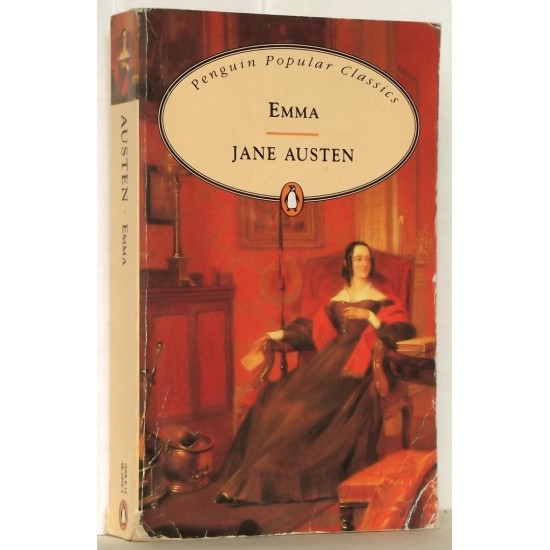On a light gray backdrop, a red and peach-colored book stands prominently. The spine of the book, visible on the upper left-hand side, features an image of a woman in the peach-colored section alongside the text "Austin" and "Emma." At the bottom, there's an unreadable word next to the distinctive Penguin Books logo.

The book cover showcases an intricate room scene dominated by shades of red. Central to the image, a woman adorned in a dark red dress sits gracefully in a chair, a red scarf draped around her shoulders. Beside her, a cabinet supports what appears to be a lamp, while an ambiguous object, possibly a cauldron, rests near her feet. The room is furnished with a dark red carpet and various pieces of light red furniture.

At the top of the cover, an oval shape, outlined in gray and black, frames the words "Penguin Popular Classics" in a peach-hued space. Below a small orange line, the title "Emma" and author "Jane Austen" are inscribed, centered within the oval. The Penguin Books logo is also centered at the bottom of this oval, providing a classic touch to this detailed and visually engaging design.